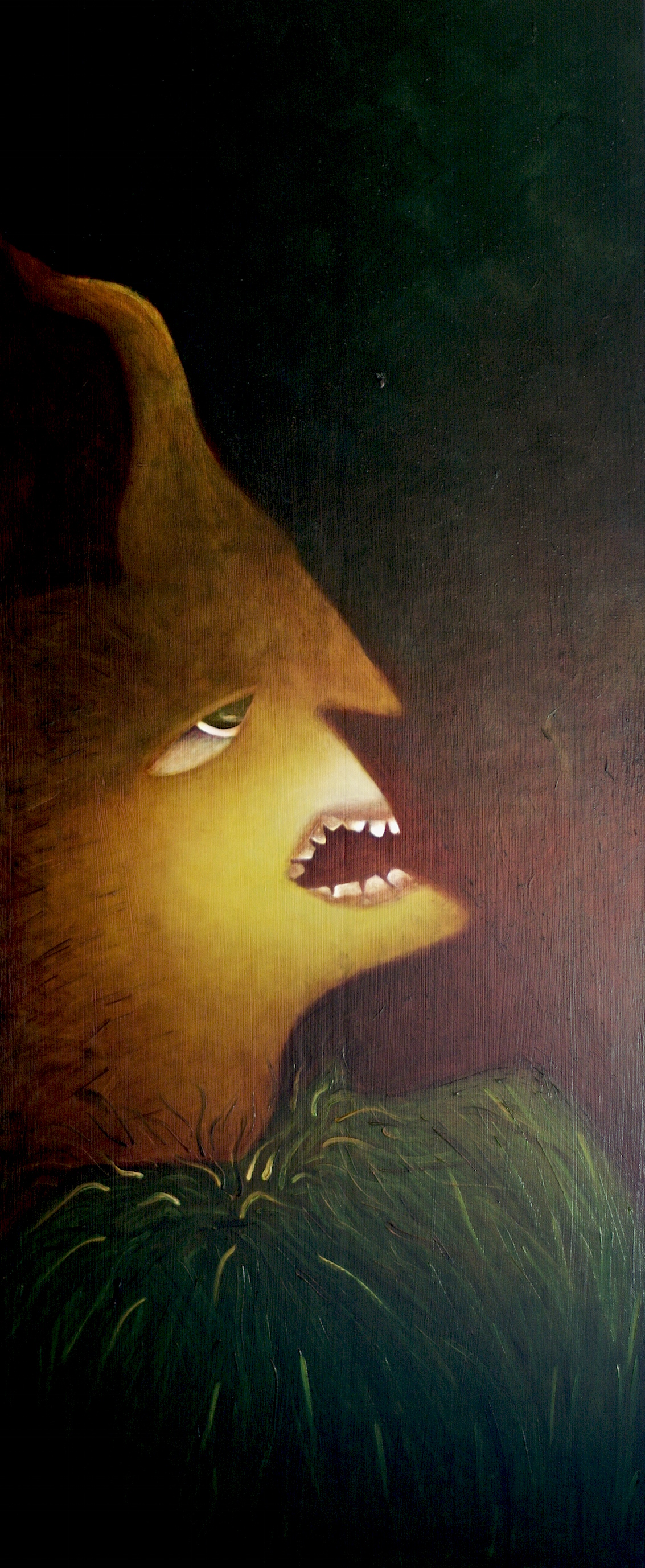This abstract painting captures a creature that resides within a dark maroon background with some greenish wisps at the top. The creature is positioned on the left half and bottom part of the image, illuminated by a light source that highlights its bizarre form. The creature's main body is green, resembling grass or weeds, with a spiky texture interwoven with yellow and dark strands.

Protruding from this green body is a highly detailed head that could be perceived as both monstrous and alien. The face is primarily a darker yellow, transitioning to a darker brown on the upper half of the head. The head itself is long, rounded, and somewhat squared with a pronounced pointy chin and a prominent, pointy nose. The creature's mouth is open, showcasing numerous glowing white teeth, giving it an aggressive or threatening appearance. The eye is large, dark green with a white background, adding an eerie focal point to the face.

One distinctive feature is a horn extending from the top of the head, contributing to the creature's otherworldly appearance. The painting deftly balances the creature's unsettling features with abstract elements, using contrasting textures and colors to create a visually striking and thought-provoking piece.